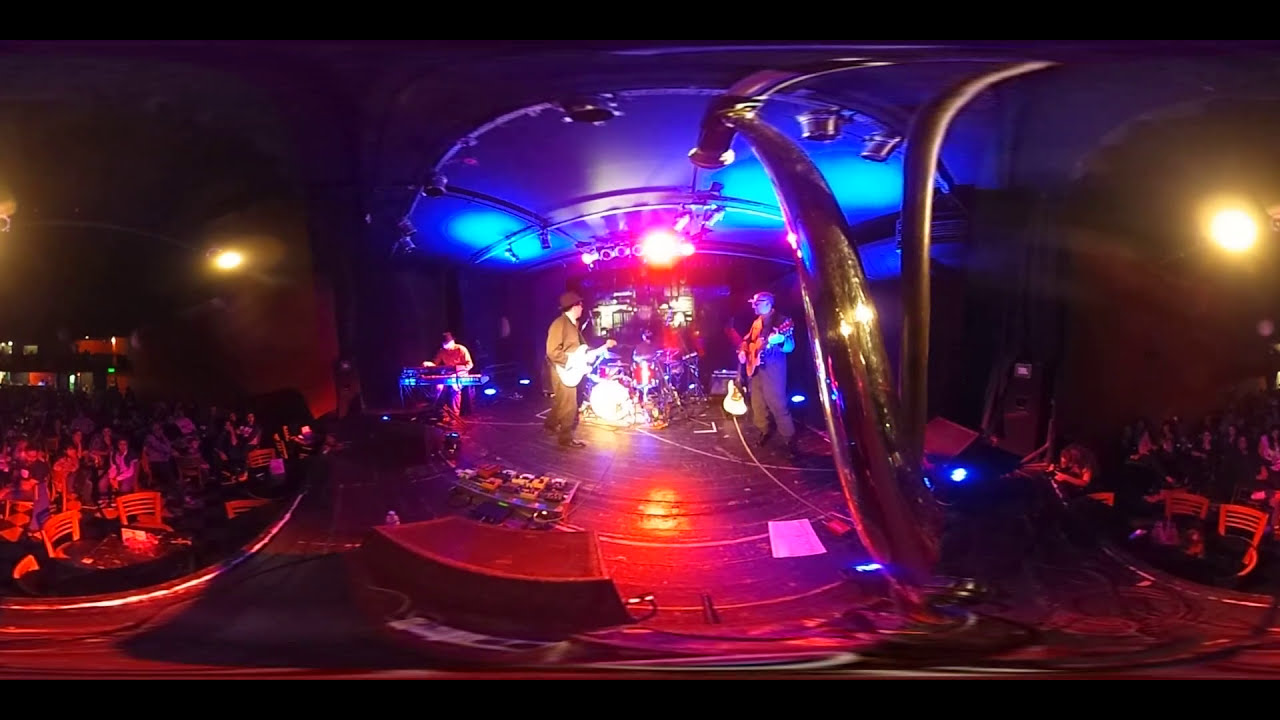The image depicts a dark, indoor concert scene with a wide, horizontal, and rectangular frame, bordered by thin black stripes across the top and bottom. Positioned in the middle of the picture is the stage, well-lit with blue and red spotlights illuminating the performers. The band members are arranged in a circle at the center of the stage. On the left, a musician in a red outfit plays a keyboard lit with blue light. To his right, a guitarist dressed in black with a black hat and white guitar looks back at a drummer in dark clothing playing a blue drum set. Another guitarist, possibly a bassist, stands on the far right, also clad in black with a dark hat. 

The stage itself features various instruments and equipment, including a black microphone with a silver head, a few steps, cables, and connections in yellow, red, black, and blue, and several black speakers. Three yellow lights enhance the stage illumination further, along with overhead blue lights against a whitish ceiling directly above the stage area.

In the audience, seated on both sides of the image, viewers watch the performance. The left side of the crowd appears in mostly gray or white clothing, while the right side is dressed in darker hues. The seating area includes brown wooden chairs and tables with black tops that seem to have a mirrored surface. The audience is moderately lit by ceiling lights, reflecting a focused and engaged atmosphere as they enjoy the musical performance happening before them.